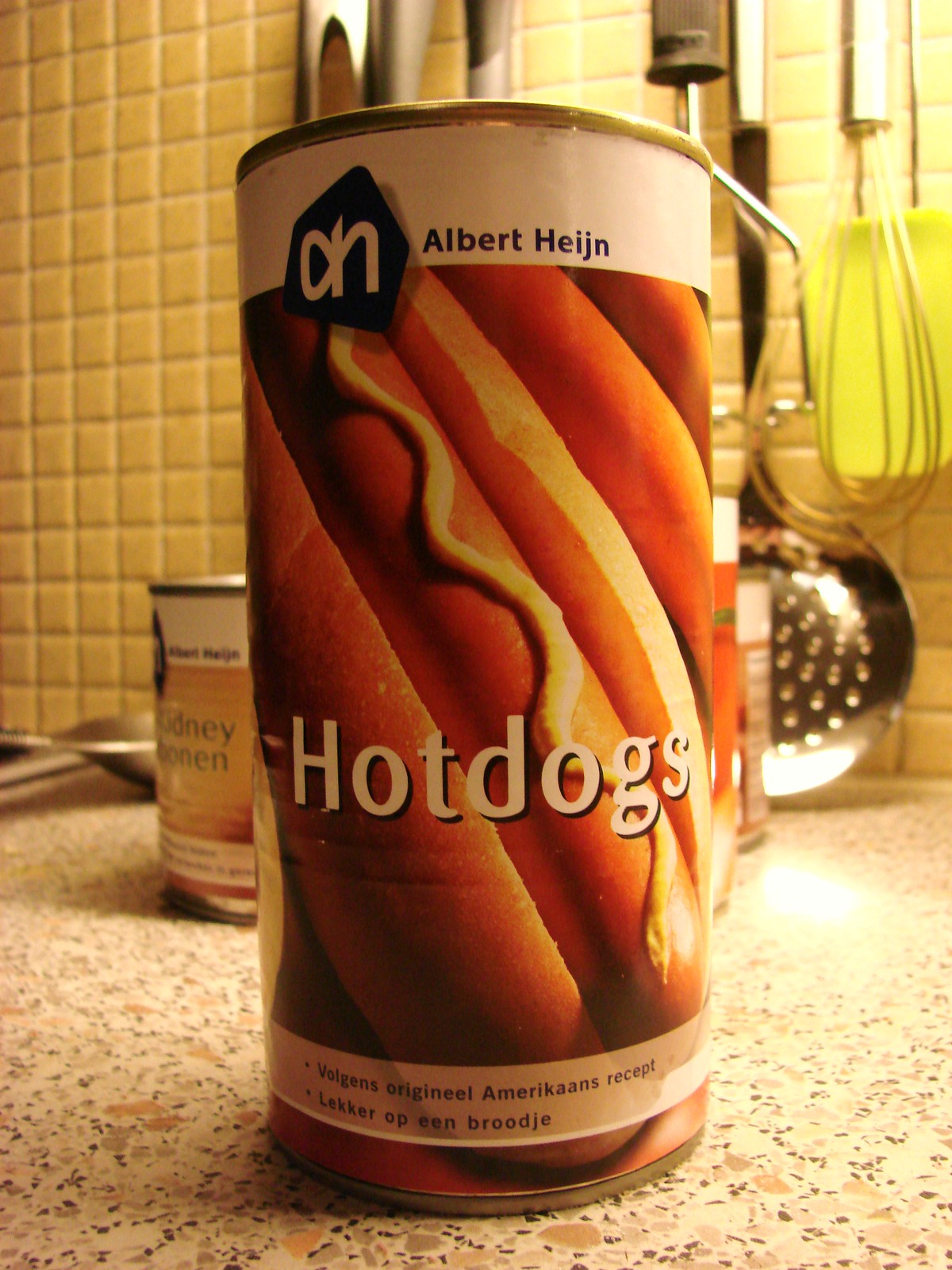The image features a can of hot dogs placed on a granite countertop that exhibits a black and white speckled pattern. The can's top is white, bearing the brand name "Jose," and includes the label "Albert, Asian." In the middle section of the can, a vibrant illustration displays several hot dogs adorned with mustard. Additionally, the can's other half includes a depiction of kidney beans in a saucy mixture, possibly suggesting a recipe idea. The background of the scene is composed of a tiled wall, providing a neutral backdrop. On the right side of the image, a whisk and a perforated ladle are visible, adding a touch of culinary ambiance to the setting. A hint of a yellow spatula is also noticeable in the backdrop, further enriching the kitchen-themed context.